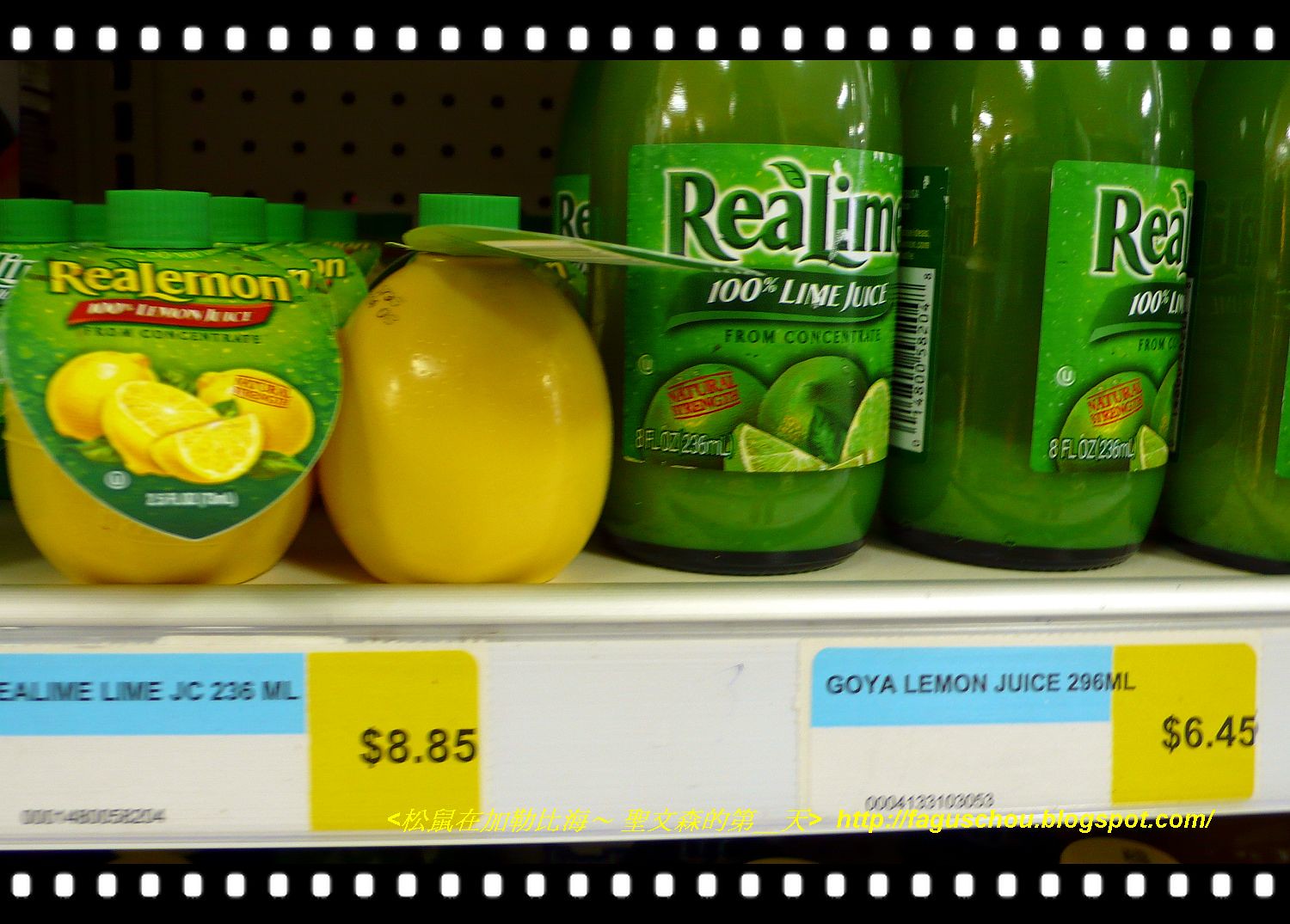This detailed image captures a close-up of a white metal shelf in a retail store, stocked with various juice products. At the bottom left of the shelf, clearly marked price labels reveal the positioning and pricing of each item. The leftmost item is a yellow, lemon-shaped bottle labeled "Real Lemon," featuring a green cap and a vivid label with "re al lemon" stylized text. The label highlights 100% lemon juice from concentrate with yellow lemon imagery against a green background. Adjacent to this, a taller green plastic bottle branded "Real Lime" displays "100% lime juice from concentrate" along with imagery of green limes. Both products have corresponding shelf tags beneath them. The "Real Lime" tag reads "real lime lime JC 236 ml" on a blue section with a blurred white UPC code area, priced at $8.85 on a yellow square. To the right of these is a bottle of "Goya Lemon Juice," distinguished by its blue-teal background on the label and priced at $6.45. Each shelf tag includes specifics about the product, followed by a series of numbers which appear to be UPC codes, although they are too blurry to discern. The entire image is bordered by a black frame with repeating white squares. Additionally, there is a faint watermark featuring Chinese characters and an English URL at the bottom of the image.